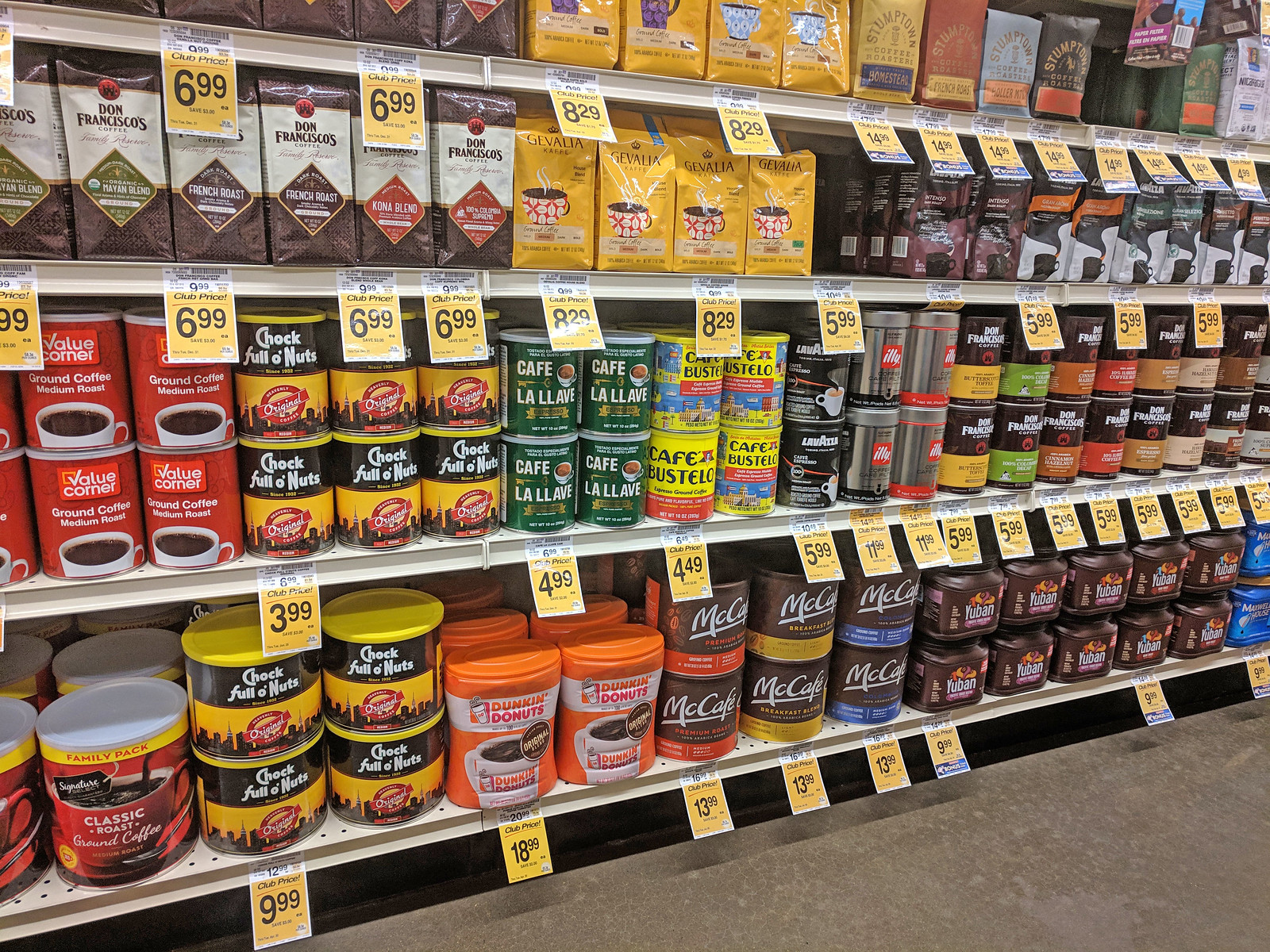This is an image of a coffee display within a grocery store aisle featuring four shelves brimming with a variety of coffee products. The bottom shelf holds larger canisters of well-known brands such as Chock Full o’ Nuts, Dunkin' Donuts, and McCafe, each priced at $9.99, $18.99, and $13.99, respectively. Moving up to the second shelf, it is lined with medium-sized containers of assorted coffee types. The third shelf houses a collection of medium-sized coffee bags, showcasing brands like Café Bustelo and Lavazza in different vibrant packaging colors like green, purple, and brown. The topmost shelf exhibits smaller bags of coffee, prominently featuring yellow Gevalia bags, alongside colorful Stumptown bags in shades of red and brown. Don Francisco and various other brands also make an appearance with blends like French Roast and Kona Blend. The display is organized with white shelf separators, and the price tags are visible below each product, indicating various prices such as $5.99, $6.29, and $8.29. The grey-toned floor adds a neutral backdrop to the colorful and diverse array of coffee products.